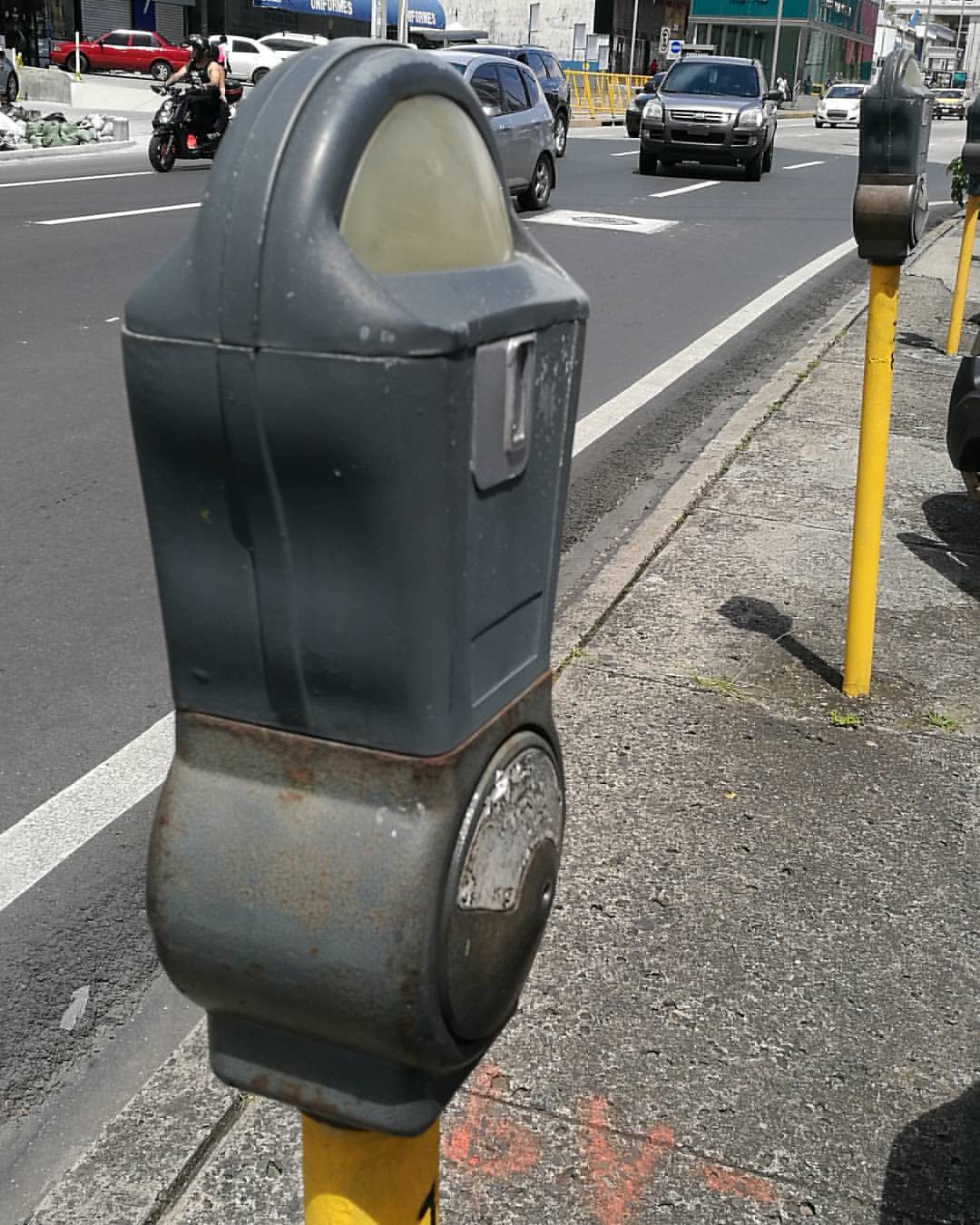The image captures a vibrant city street bustling with activity. Dominating the foreground is an aged parking meter, standing on a sidewalk that stretches alongside the road. The parking meter, perched on a yellow pole, is notably old and worn-out, with significant rust covering both its dark gray top and lighter gray body. The glass covering the coin slot and timer is foggy and dirty, making it impossible to read the time left. The sidewalk itself appears decrepit, with visible cracks, debris, and faded paint markings. Despite the absence of parked cars by the meters, the street teems with traffic, including an SUV, various cars, and a motorcycle moving towards the viewer. The chaotic atmosphere underscores the city's relentless pace.